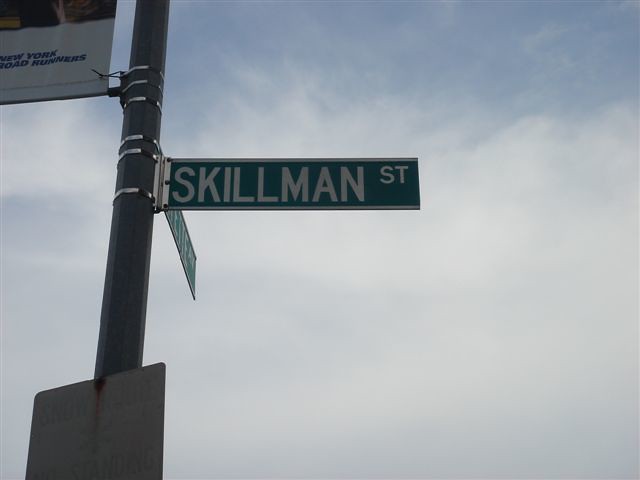In this image, we see a pair of street signs mounted on a tall, metal pole positioned on the left side of the frame. The most prominent sign, clearly visible, reads "Skillman ST" in white letters against a green background, accented by a white trim. The second sign is oriented towards the left, making it difficult to decipher the street name due to the angle. Additionally, below these signs, there's a faded sign that seems to read "snow," although the text is barely legible. The street signs are oriented in different directions, indicating multiple pathways or streets intersecting at this location.